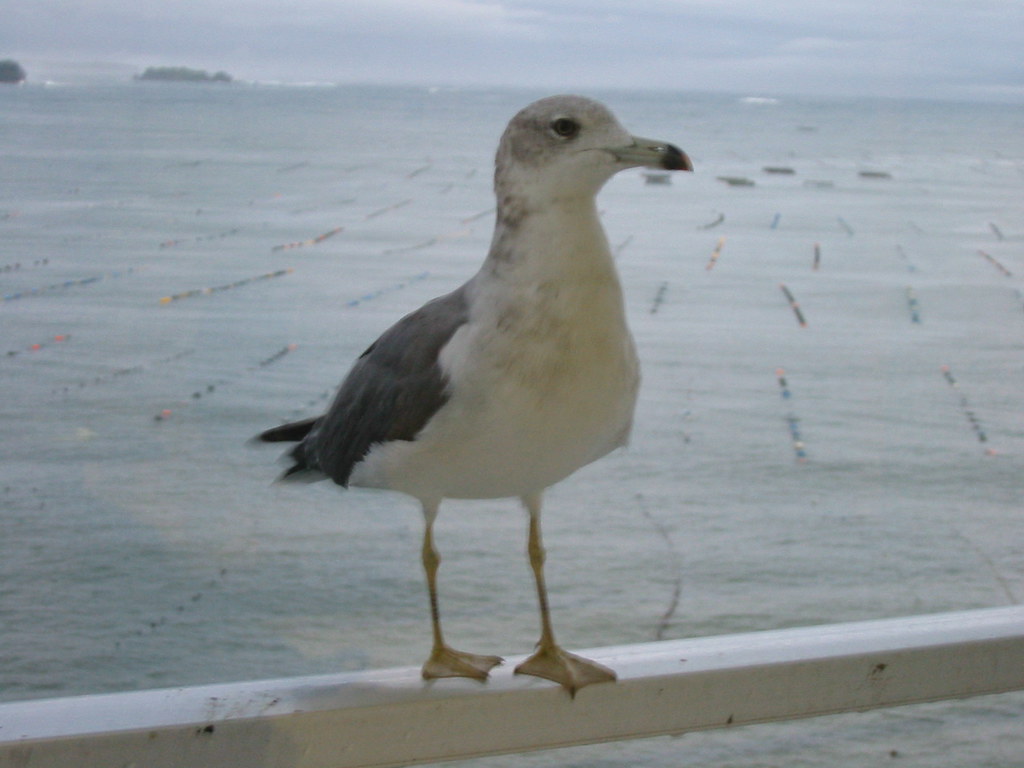This is a detailed photo of a seagull standing on a white rail above a water area. The bird is facing the viewer but turned slightly to the left, obscuring the left side of its head. The seagull, approximately a foot tall, has a white body with black wings accented by a touch of gray. It features dark eyes and a gray beak with a black tip. Its webbed feet are bright yellow. The background reveals a distant land under a very cloudy daytime sky. The water below the seagull displays colorful strips of yellow, red, blue, and green.